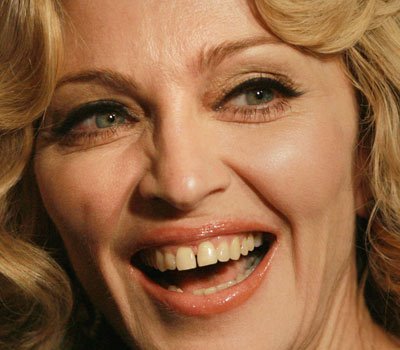In this detailed and contemporary close-up photograph, we see the iconic pop star Madonna as an older, mature adult. She is captured smiling broadly with an open mouth, revealing both her top and bottom teeth, and a signature gap between her front teeth. Her blonde, wavy hair frames her face, cascading down but mostly out of the frame. Madonna's eyes, a striking green or hazel color, look off to her right, adding to the warmth and expressiveness of her smile. Her high cheekbones are highlighted by the lighting, which illuminates the right side of her face while leaving the left slightly shadowed. She wears shimmery eyeshadow, thick eyeliner, and mascara that accentuate her thin eyebrows, matching the color of her hair. Her lips are adorned with light red or pink lipstick, complementing her jubilant expression. Visible wrinkles around her eyes, nasal labial folds, and a slightly wrinkled neck reflect her age while still capturing her timeless charm and energy.